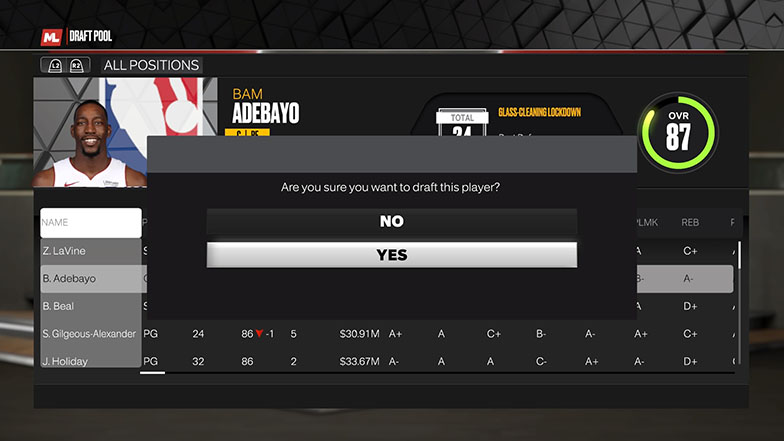This is a detailed screenshot of an NBA draft pool interface, which may be part of a gambling site or a drafting platform. 

In the upper left corner, there is a logo featuring an "M" within a red box. To the right of this logo, "DRAFT POOL" is prominently displayed in uppercase white lettering against a black background. 

Below this header, instructions "L2 R2 All Positions" are visible. Then, a photograph of an NBA player appears, identifiable by the NBA logo in the background. The player is Bam Adebayo, with his first and last name displayed to the right of his image. 

Below Bam's name, there are several yellow boxes with unreadable text. Further to the right, it reads "Total: 24 Glass Cleaning Lockdown." 

Adjacent to this, "OVR 87" is denoted, surrounded by a light green circle highlight that runs from the 12 o'clock position to around 10 o'clock. 

Overlapping this content is a pop-up window that asks, "Are you sure you want to draft this player?" with options to select "No" or "Yes." In the background, additional stats about various other players are also visible, providing a comprehensive overview of the draft pool.